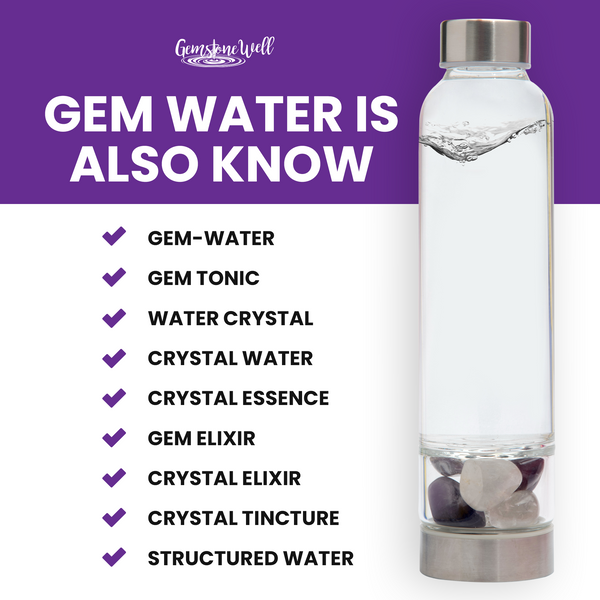The image is a detailed advertisement for a product called "Health Water" from the brand Gemstone Well. The main feature of the ad is a clear glass water bottle, which is tall and slender with a gray cap at the top and a metallic base at the bottom. Inside the bottle, gemstones are visibly placed at the bottom, separated from the water above. The design suggests that the water interacts with the gems, possibly providing some touted benefits.

At the top of the image, there is a purple banner stating "Gemstone Well," followed by confusing text that reads, "Gem water is also no." Below this, there is a list of various terms that are presumably synonyms or alternative names for gem water, each accompanied by a purple check mark. The terms listed are: gem water, gem tonic, water crystal, crystal water, crystal essence, gem elixir, crystal elixir, crystal tincture, and structured water. 

The intent of the ad appears to be to inform potential customers that gem water can go by many different names, though the meaning and benefits are not well explained, making the advertisement somewhat confusing.